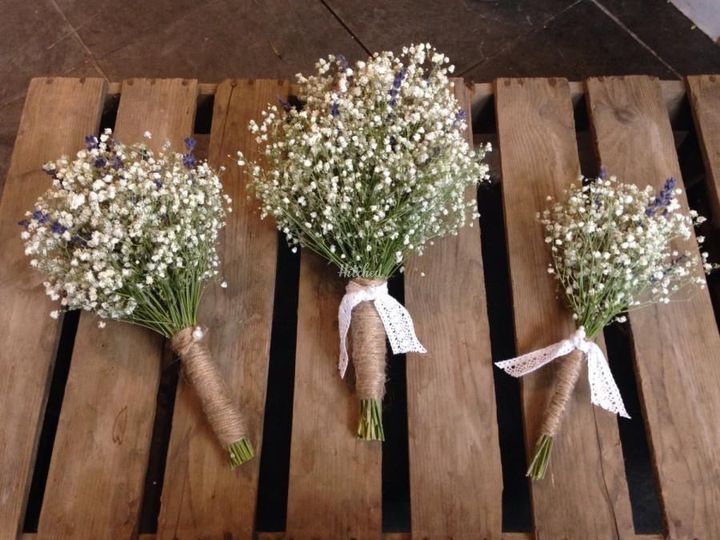This color photograph, taken in daylight, features three bouquets of baby's breath flowers placed side by side on a rustic wooden pallet composed of several panels with vertical cutouts. The flowers, predominantly tiny white buds resembling clouds or snowflakes, are bundled together, each glints of conical purple blossoms interspersed. The stems are partially visible and wrapped in brown twine, with the middle and right bouquets adorned with additional white lace bows. The wooden surface rests on a dark brown, rough-textured tiled floor. Notably, the bouquets vary in size, with the left being medium, the center the largest, and the right the smallest, adding a sense of organized simplicity to the arrangement.